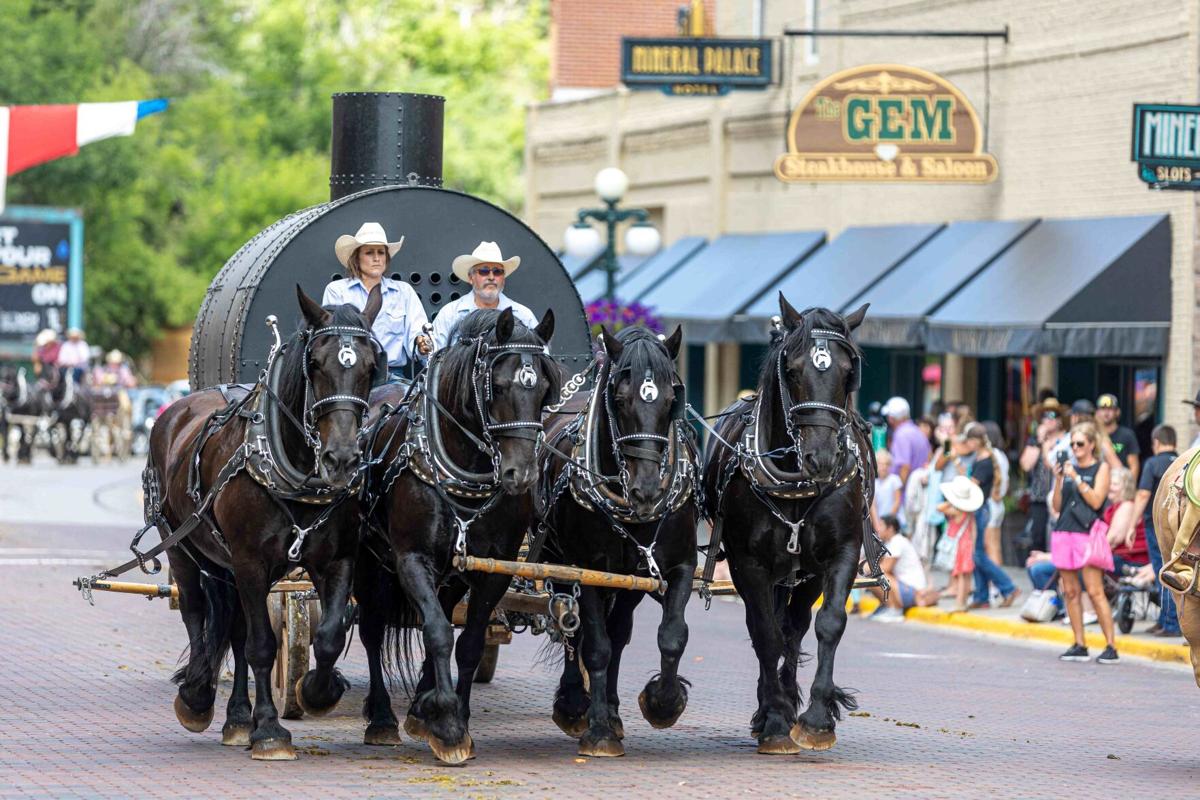In this vibrant parade scene, four majestic draft horses, possibly Frisians or Studebakers, are majestically pulling a large, black barrel-shaped smoker, which intriguingly features a smaller barrel positioned on top, possibly serving as a chute. The horses, in full harness with gleaming brass and silver, are moving down a modern city street with yellow curbs. The street is lined with buildings, featuring signs such as one partially reading "Gem" and another with "Palace" in its name, suggesting a setting in a western state with a nod to historical reenactment.

Guiding the procession are two serious-looking drivers—a man and a woman—both clad in white long-sleeved button-up shirts and white or beige cowboy hats, adding to the old-timey ambiance of the event. The parade atmosphere is enlivened by a large crowd of spectators, many of whom are eagerly taking photographs, capturing the nostalgic spectacle of this modern-day homage to a bygone era.